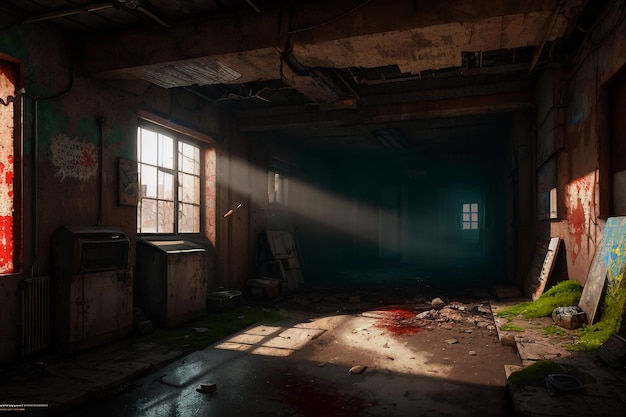The image, which could be a photograph or a painting, showcases a dilapidated and dimly-lit interior of an abandoned building, possibly a studio or factory. This space features three windows, with the one on the left side allowing beams of sunlight to penetrate the room, illuminating the dust particles floating in the air. The room is in a state of severe disrepair; the ceiling appears to be collapsing, and the floor is littered with various debris and detritus.

There are numerous items scattered around, including old, rusted materials, a wooden pallet, and an abandoned canvas. The walls, originally dark red, now have a faded clay color with patches of peeling paint. On the right-hand side against the wall, greenery or moss has started to grow, adding to the sense of neglect. Some old paintings, mostly spattered with red, blue, and green paint, lean against the wall. A Ouija board drawing in black text can be seen next to the left window, possibly on a bacteria-shaped board.

On the floor, there are red streaks and white chemical stains, giving the impression of an old, chaotic workspace. The air conditioning units near the left window appear aged and unused. The room is overall very dark, save for the single stream of sunlight that casts a warm glow on the floor and canvases, creating a striking contrast in the image.